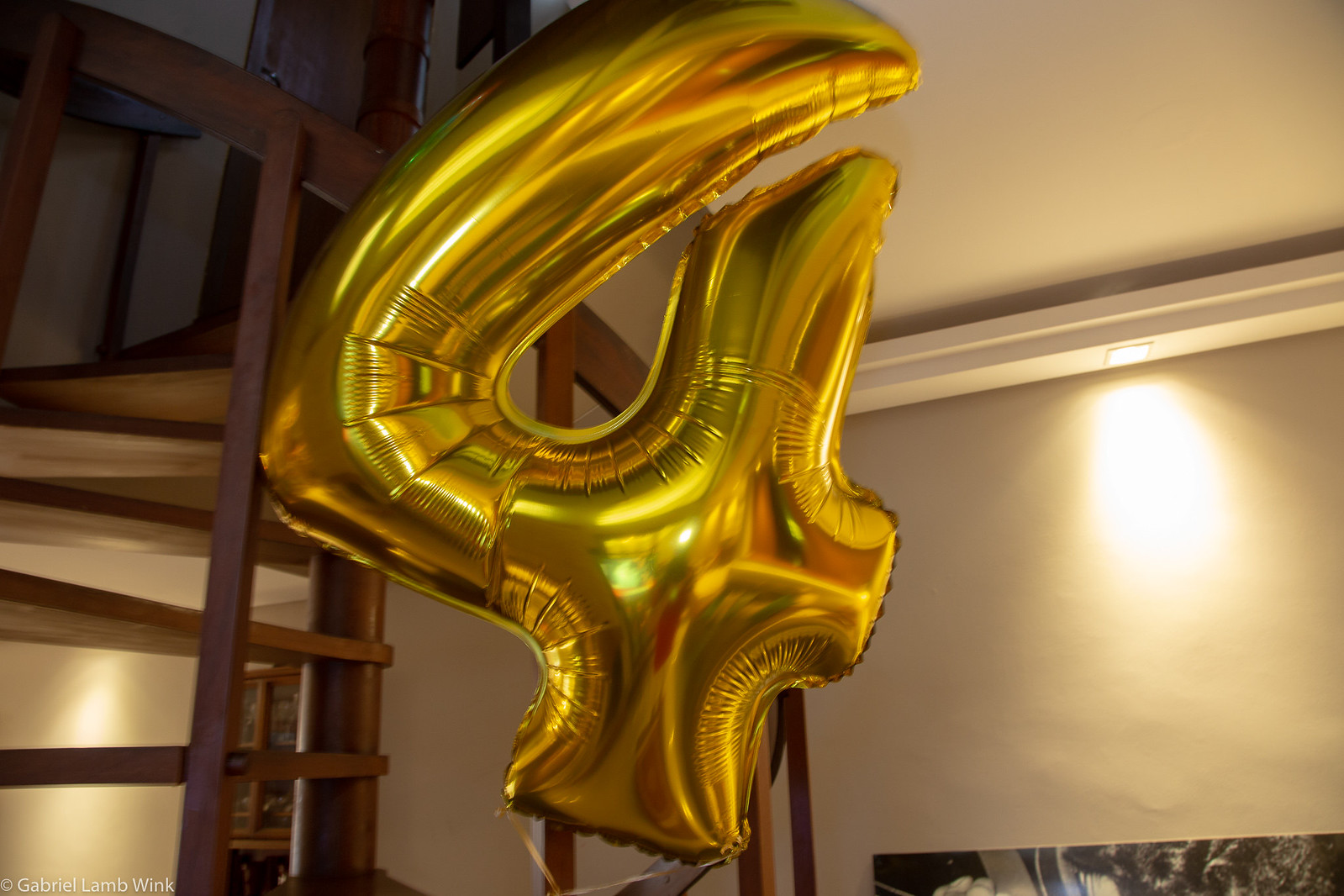This indoor color photograph captures a helium-filled, golden metallic balloon shaped like the number four, prominently floating and slightly reflecting its surroundings. The balloon is positioned near a brass spiral staircase, which features brass handles and lighter brass or metal steps that wind up to a second floor, partially visible at the top left of the image. A white wall with a shelf and a recessed light underneath shines down on the scene to the right. The wallpaper behind is illuminated, appearing as white paint. In the lower right corner, the partial edge of an artwork or TV is visible. The ceiling and walls are white, and a chair is spotted to the left of the balloon. Additionally, the bottom left corner of the image contains a copyright symbol with the text "Gabriel Lamb Wink" in white.